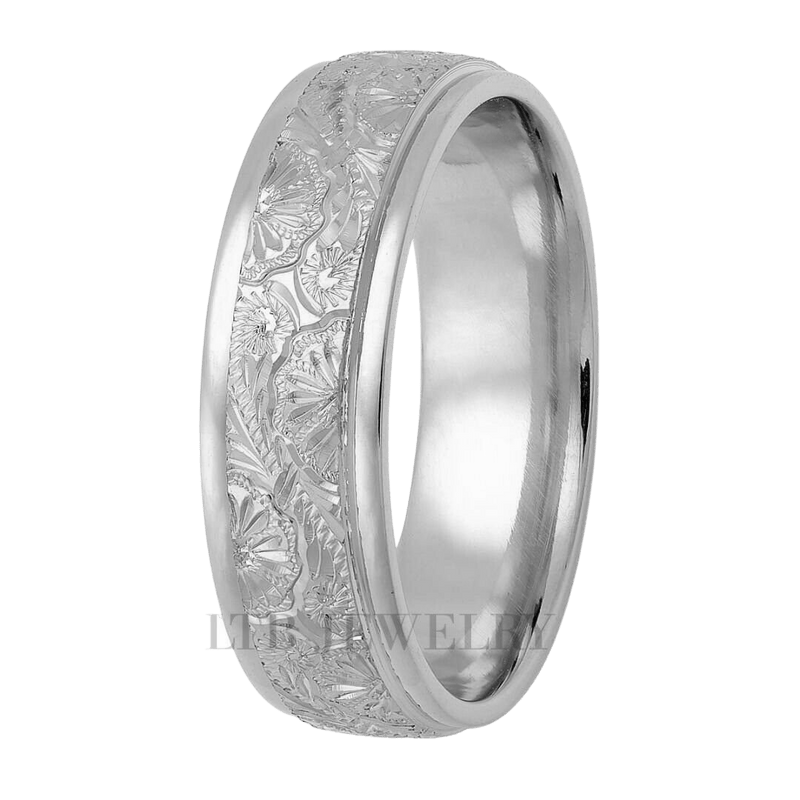The image depicts a ring viewed from an angle that showcases its side profile. The ring itself is devoid of gems, which accentuates its elaborate band design. The band features intricate floral patterns, creating a delicate and flowing aesthetic. On the left side of the visible portion, there is a half-flower design with adjacent leaves, forming a bumpy circle along the edges. Interspersed between these floral elements are a series of lines that converge into a prominent flower at the top. The design gracefully curves from the top to the bottom right, suggesting a continuous and repeating floral motif. The foreground displays the inscription "LTEB Jewelry," signifying the brand or maker of the ring.